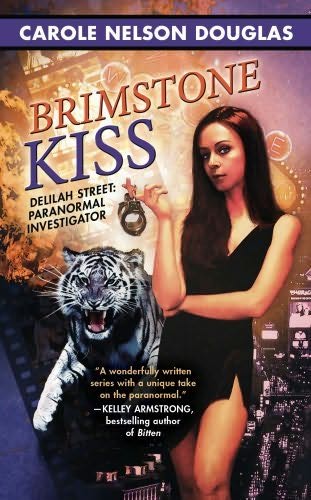This image features the front cover of a book or a promotional poster for a series. At the top, a purple bar with thick black borders holds the white, all-caps text "CAROL NELSON DOUGLAS." The background displays a fiery surface adorned with shiny objects, creating an intense and dramatic setting. The title of the book, "BRIMSTONE KISS," is written diagonally in all-caps, with "BRIMSTONE" in orange and "KISS" in purple. Below the title, it says "Delilah Street Paranormal Investigator" in black font. To the right, a striking woman with long dark hair and light skin is depicted wearing a short black dress. She is holding a pair of handcuffs in her left hand. Beside her, a roaring white tiger appears to be charging, adding to the dynamic and supernatural theme. In the background, there is a faint view of a city skyline, completing this engaging and vivid scene.